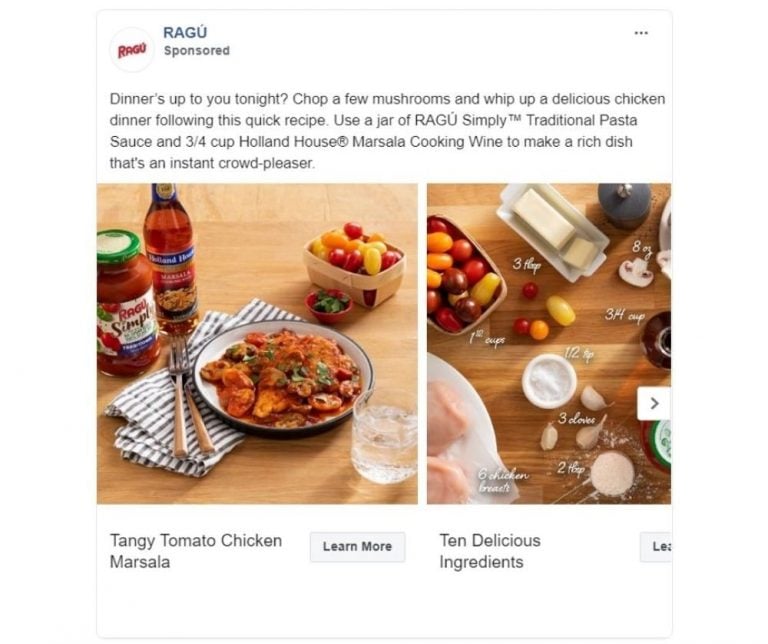The image is a sponsored social media post, possibly on Instagram, although it is unclear due to cropping and significant artifacting. The post is set against a predominantly white background and is published by Ragu, as indicated by their circular logo avatar. On the far right, three dots offer post options. The image itself is horizontally scrollable.

The main photo features a plate of pasta topped with red sauce and large chunks of eggplant. This is set on a light wood table adorned with cherry tomatoes in varied colors and some herbs in small baskets. Additionally, there is a bottle of an indiscernible product and a jar of Ragu sauce included in the frame. To the right of this image is a white arrow indicating the ability to scroll for more content.

The subsequent image is titled "Ten Delicious Ingredients" and continues the light wood table theme. It displays an assortment of ingredients, including multicolored cherry tomatoes, salt, garlic, chicken, mushrooms, and butter, arranged with measurements. There are also several unmarked bottles with a note indicating "3/4 of a cup" next to some of the ingredients. This composition showcases the various components presumably needed to prepare a dish highlighted by Ragu.

Overall, the post promotes a culinary experience with Ragu products through visually appealing, detailed presentations of ingredients and the finished pasta dish.